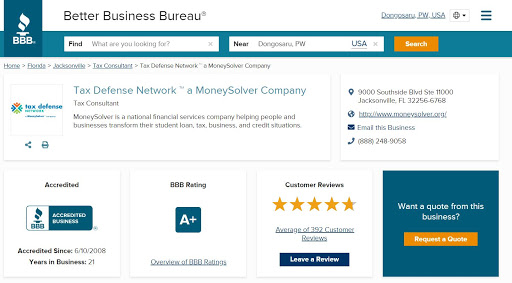This screen capture is from the Better Business Bureau (BBB) website. In the top left corner, the BBB logo is displayed, featuring a white torch with white flames. The top right corner has the text "Dungasaru PW USA." Below the BBB text, there is a search bar labeled "Find what are you looking for," and to its right, another search bar labeled "Near Dungasaru PW USA," adjacent to a yellow search button.

Below these elements, the page showcases navigational blue hyperlinks: "Home," "Florida," and "Jacksonville," followed by "Tax Consultant." Further to the right, in gray font (not a hyperlink), it says "Tax Defense Network, a Money Solver Company."

Beneath this text, a detailed section advertises the Tax Defense Network as a "Tax Defense Network, a Money Solver Company." To the left of this advertisement is the Tax Defense Network icon. The address listed is 9000 Southside Boulevard, Suite 11000, Jacksonville, Florida. The website link is displayed as "www.moneysolver.org," followed by the prompt "Email this business."